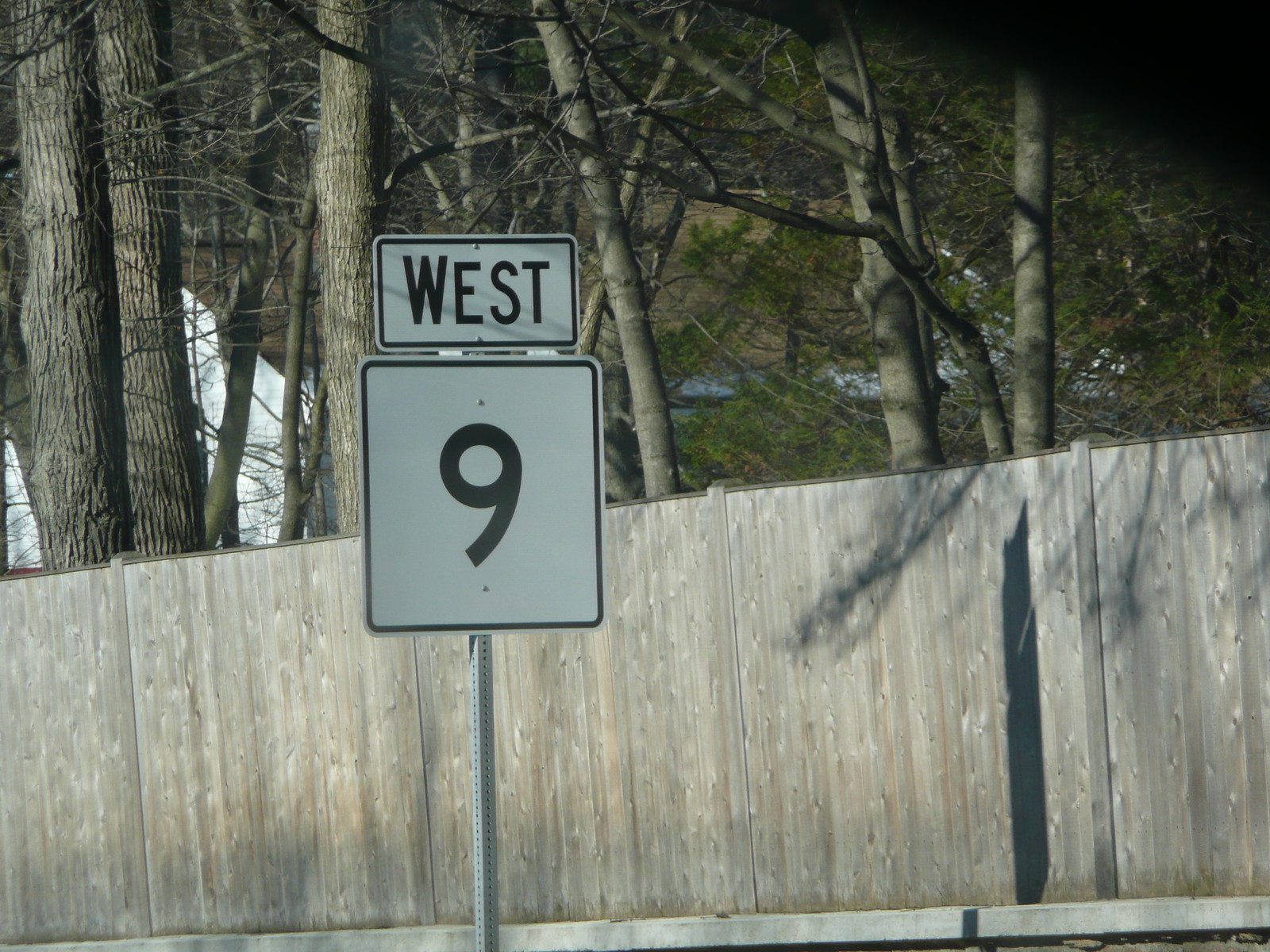In this image, the focus is on a sign. The back of the sign is white, prominently displaying a large black number "9". Just above this white square sign, there is a rectangular white sign with a black outline, containing the black text "WEST". The background features a tall, light brown privacy fence that stretches continuously from the left edge to the right edge of the photo.

Behind the fence, there are several tall trees. Their thick, rough bark is a lighter shade of brown. On the left, two thicker trees appear, while in the center, there is another thick tree surrounded by thinner branches. To the right, four more trees with noticeable trunks stand out.

The ground in the background shows patches of green grass, interspersed with spots of white snow on a slight hill. In the upper right corner of the photo, a shadow covers several inches, while the shadows of the trees are also visible, casting patterns along the privacy fence.